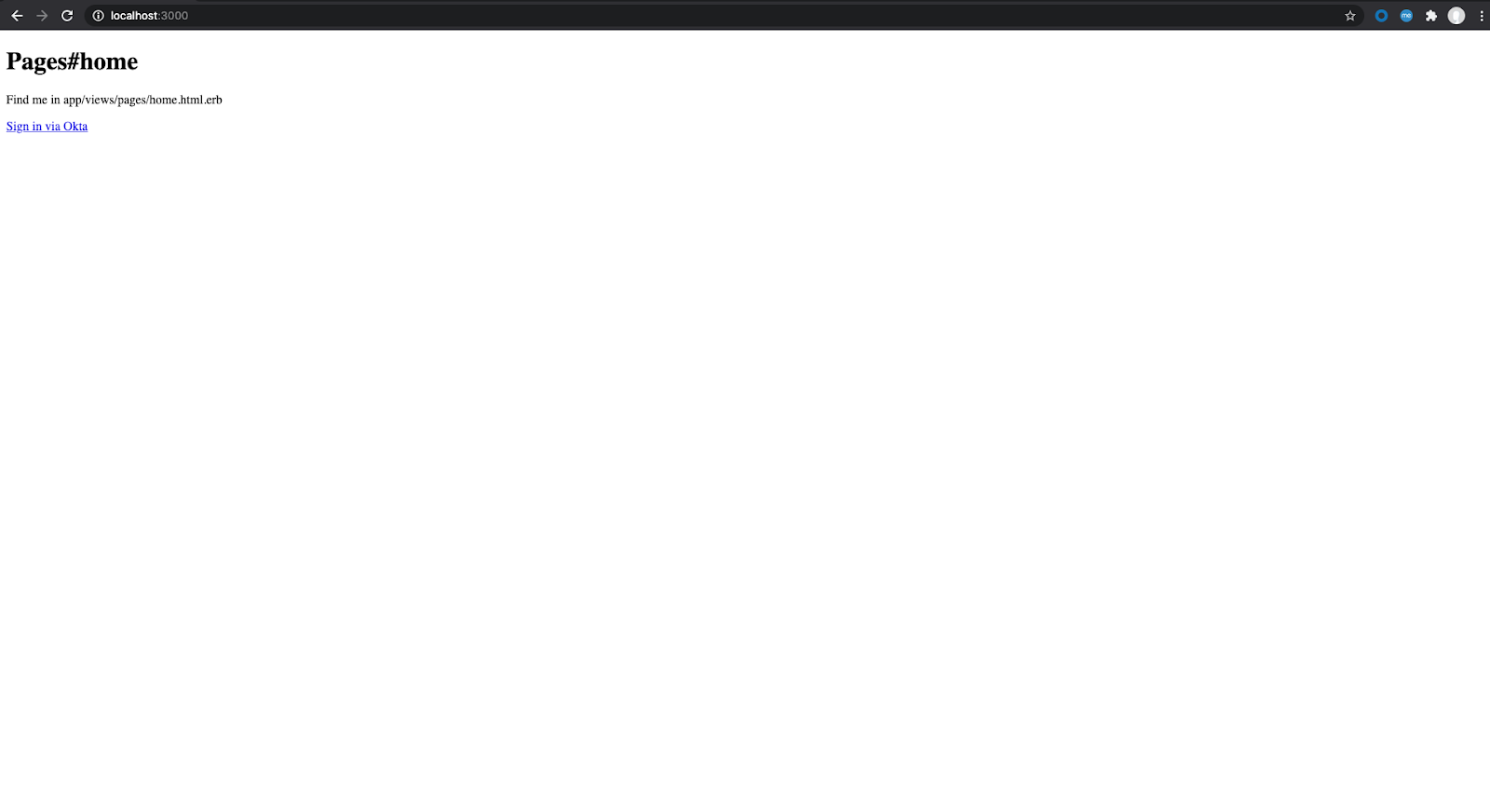This is a screenshot of a web browser displaying a minimalist web page. At the top of the browser, there is a black toolbar featuring white icons for navigation: a back arrow, a forward arrow, and a refresh arrow. This toolbar also contains a text area for the website address, which is indecipherable due to the low-quality, pixelated nature of the image. On the right end of the toolbar, there is a five-pointed star icon used for bookmarking, followed by additional icons, including one that resembles a puzzle piece and another appears to be a blue circle.

The main content area of the browser is largely blank, with a predominantly white background. Positioned in the upper left corner, bold black text reads "Pages #Home." Below this header, there is a subtext in standard font that says "Find me in app/view/pages/home.html.erb," which likely indicates the file path of the displayed page. Beneath this, a clickable link in blue font reads "Sign in via Chiba." The image does not contain any additional elements or content beyond what has been described.